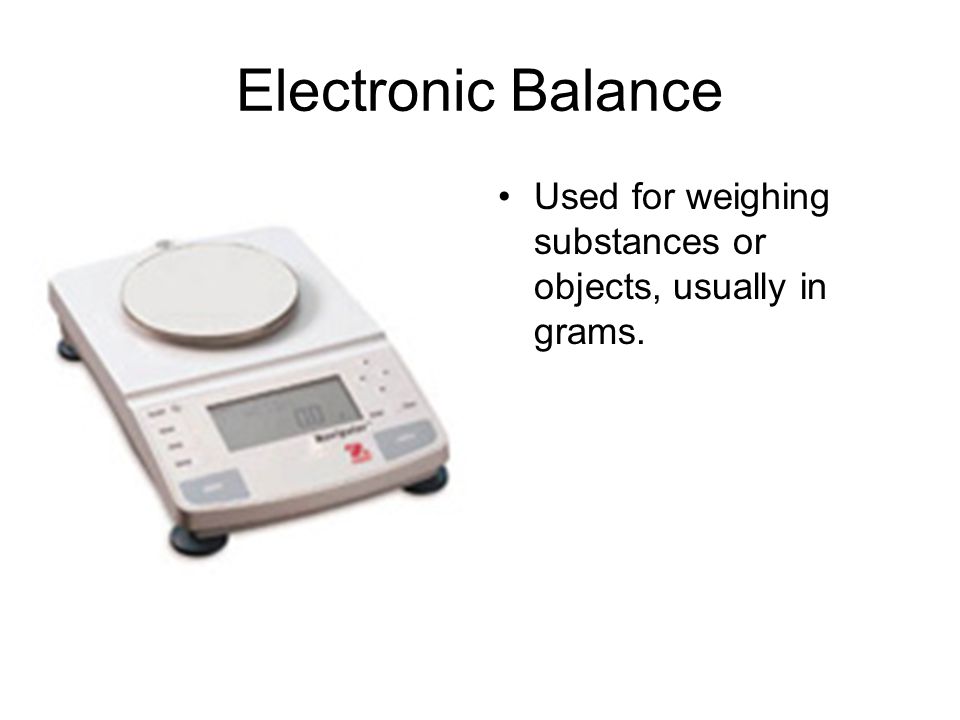The image features an electronic balance prominently positioned on the left side. The scale has a white body with a circular metal plate on top used for weighing substances or objects, typically in grams. The display is gray and shows a reading of 0.0, flanked by multiple buttons—four on the left and six or seven on the right. The scale is supported by four black circular stands resembling plastic buttons, ensuring stability. A red company logo is situated near the center at the bottom of the scale. To the right of the image, there's a bullet point paragraph that reads "used for weighing substances or objects, usually in grams." Above the scale, the title "Electronic Balance" is displayed in black font.